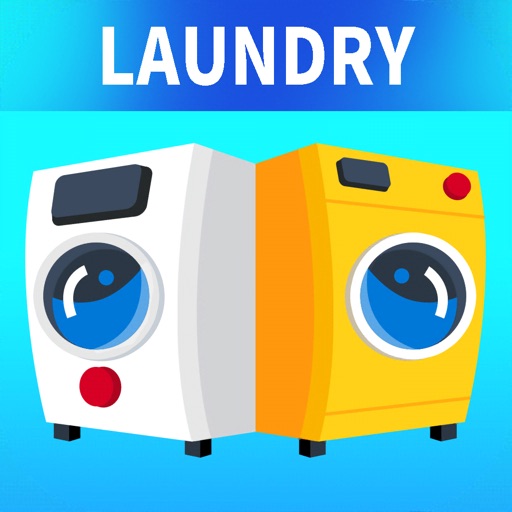The image is a cartoon illustration set against a light blue background, featuring a darker blue horizontal banner at the top. Centered within this banner, bold white letters in all caps spell out "LAUNDRY." Below this, two laundry machines are displayed. On the left is a white machine, facing slightly left, with a black horizontal control panel at the top and a large circular window in the center for loading laundry. Below the window is a prominent red button, and the machine stands on two small black feet. Beside it, angled to the right, is a yellow machine. It features a smaller black rectangular panel at the top left and a red button on the top right. Similarly to the white machine, it also has a central circular window for loading laundry and two black feet. Both machines are depicted with cartoonish detail against the light blue backdrop.